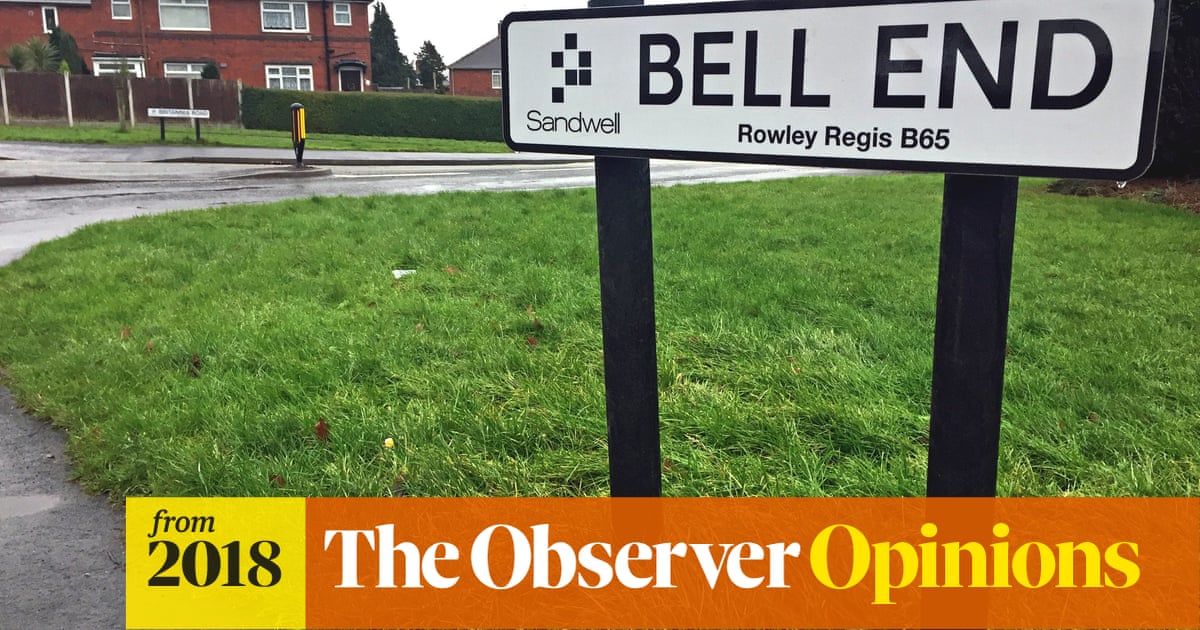This outdoor photograph prominently features a lush, green grassy area that occupies most of the scene. In the top left corner, there is a red brick building, possibly a house or another type of structure, partially obscured by various types of fencing. A wooden fence and a shrub fence are visible, along with a road running adjacent to the grassy area.

On the right side of the grassy area, a sign reading "Sandwell" is prominently displayed, with large text below it displaying "Bell End, Raleigh, Regis, D65." At the bottom of the image, a yellow box contains the text "From 2018" in black, next to an orange box that extends to the right edge of the photo. Within the orange box, the word "The Observer" is written in white text, and below it, "Opinions" is highlighted in yellow text.